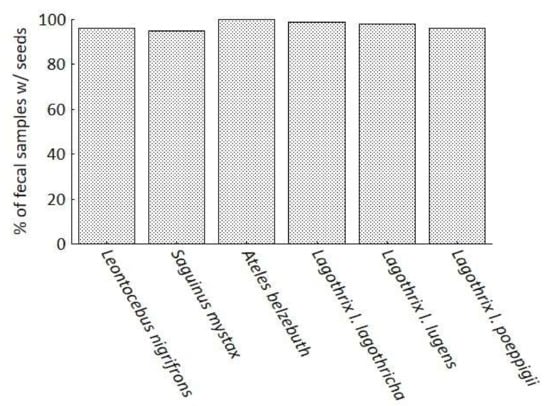The image depicts a black-and-white bar graph with bars shaded in gray, illustrating the "Percent of Fecal Samples with Seeds." The vertical axis is labeled from 0 to 100 percent in increments of 20. The horizontal axis features complex and scientific labels, including species names such as Leontopithecus nigrifrons, Saguinus mystax, Ateles belzebuth, Lagothrix lagothricha, Lagothrix lugens, and Lagothrix poeppigii. All bars are above the 90% mark, with Ateles belzebuth reaching nearly 100%, closely followed by Lagothrix lagothricha around 95%, and Lagothrix lugens slightly lower. The remaining species are also in the 90% range, indicating a high presence of seeds in their fecal samples.